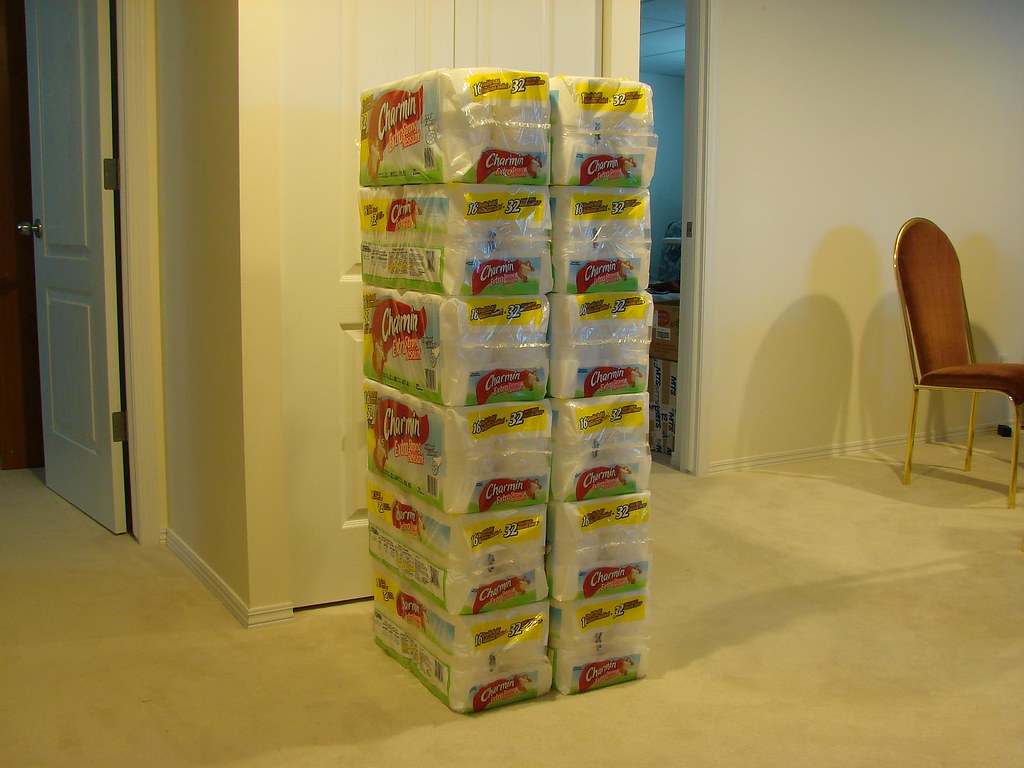This indoor photograph appears to be taken inside a home, showcasing part of a room with off-white walls and three doorways. Two of the doorways are open: the one on the left reveals a closed brown door behind it, while the one on the right leads into a walk-in closet. Positioned between these two doorways is a closed closet door. In front of this closed closet door, on the floor, are 12 packages of Charmin toilet paper, arranged in two columns of six packages each, each plastic-wrapped with the recognizable red Charmin logo. To the right, beside the doorway leading to the closet, is a rust-colored chair with a gold frame. The overall setting appears to be carpeted, contributing to the homey ambiance of the space.